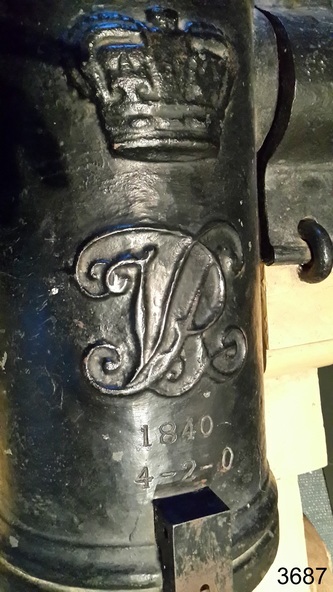This close-up photograph captures a vertical, cylindrical metal object, likely made of steel or iron and painted black or gray. The object dominates the rectangular image, extending from the top to the bottom. Beginning at the top, the piece features a molded crown design that stands out slightly from the surface. Just below this crown, the metal bears intricate, potentially calligraphic initials that resemble a decorative "V and B" or "V and R." Further down, the object is inscribed with the year "1840" followed by "4-2-0." To the side, in the upper right section, a horizontal extension suggests functionality, possibly as part of a gate or door mechanism, and includes a dark gray hook attaching to a lighter wood element. The photograph also displays the stamped numbers "3687" at the bottom right corner, adding to the detailed craftsmanship and historical context of the piece.